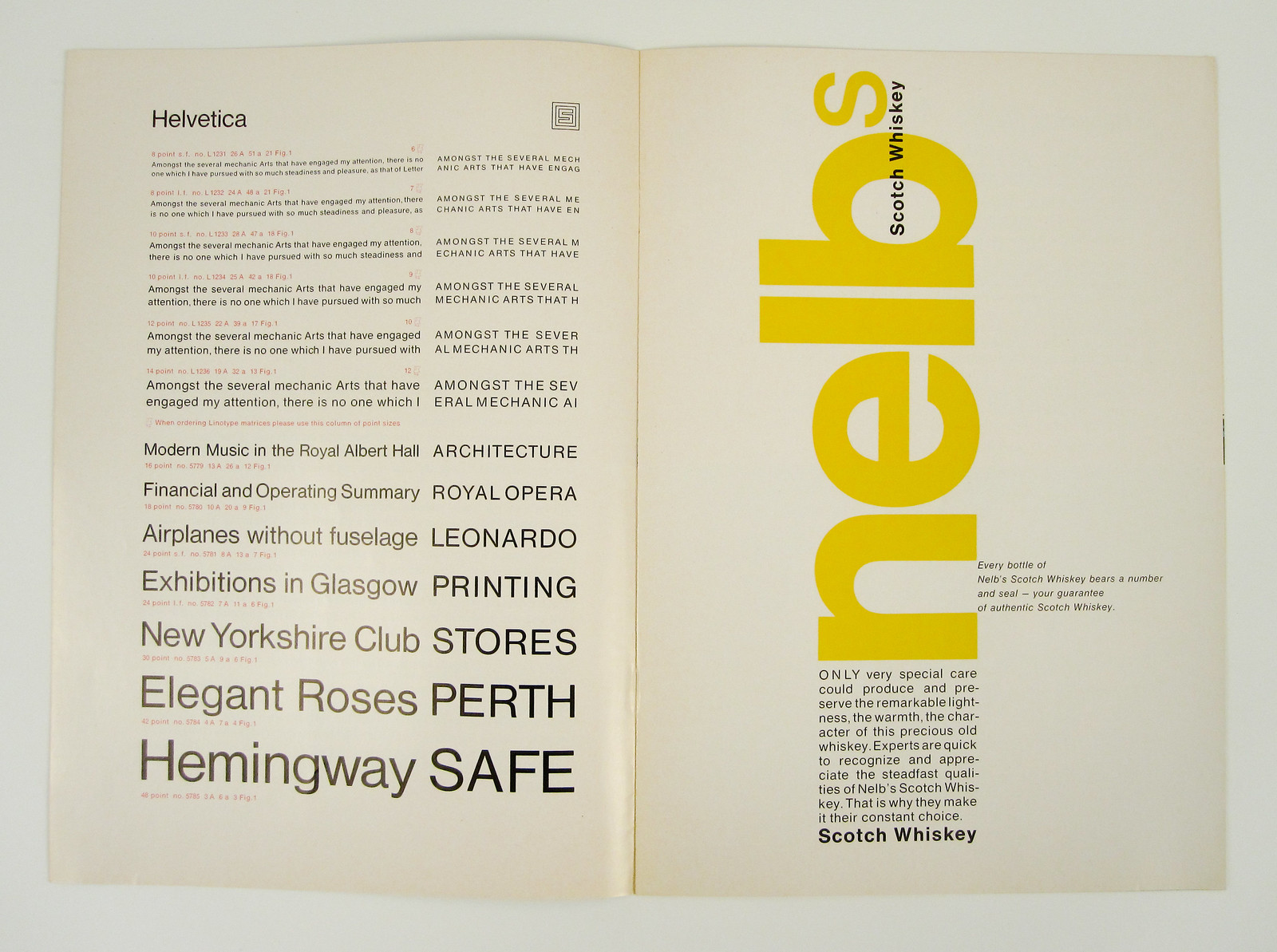This large square image features an open booklet centered against a solid gray background, which appears more like a border. The left page showcases a variety of text in Helvetica font, organized in a way that the font size increases as it progresses downward, culminating with the largest text at the bottom, stating "Hemingway Safe". Other words included on this page are "Elegant Roses Perth," "New Yorkshire Club," "Stores," "Exhibitions in Glasgow," "Printing," "Airplanes with Fuselage," and "Leonardo." Additionally, a small maze illustration is present on this page, emphasizing the typesetting and design elements.

The right page diverges slightly with a vertical arrangement of text in large block yellow letters reading "NELB," followed by a small 'S', above smaller black print that reads "Scotch Whiskey." Below this, a descriptive paragraph praises the quality and care involved in producing the whiskey, emphasizing its remarkable lightness, warmth, and character. It further affirms that experts consistently recognize and prefer NELB's Scotch Whiskey, making it their constant choice. This segment concludes with "Scotch Whiskey" in larger bold letters at the bottom.

The entire spread seems to serve as an illustrative example of different font types, typographic design layouts, and commercial printing, with a focus on both Helvetica font variations and a promotional depiction of NELB's Scotch Whiskey.